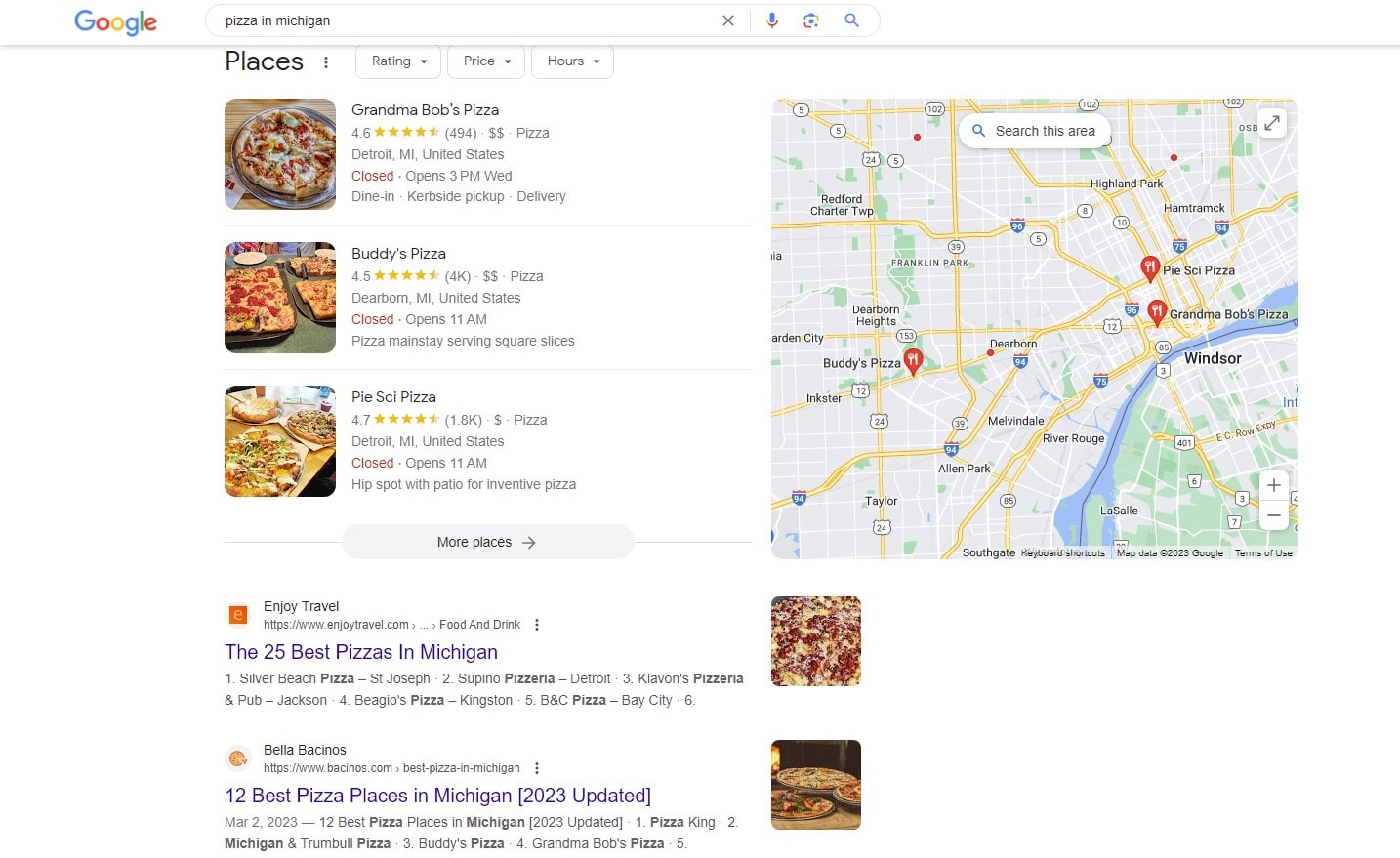The image features a Google search interface against a white background. At the top, "Google" is displayed in its distinctive multicolored logo. Below it, there is an oval-shaped search box outlined in gray. Inside the search box, the term "Pisa in Michigan" is typed in a black font. To the right of the search box is a gray "X" for clearing the text, and a blue microphone icon for voice search.

Beneath the search box, there are search results for pizzerias in Michigan. The first result is "Grandma Bob's Pisa," which has a rating of 4.6 stars based on 494 reviews. It is located in Detroit, Michigan, and listed as offering a $2 size pizza. The pizzeria is marked with a red "closed" status and indicates that it opens at 3 p.m. on Wednesdays. It offers dining in, curbside pickup (spelled as "kerbside"), and delivery services.

The second result is "Buddy's Pisa," with a 4.5-star rating from 4,000 reviews, located in Dearborn, Michigan. It is also marked as "closed" but notes that it opens at 11 a.m. The description mentions its location on Main Street and features 7 square slices of pizza.

The third result is "Pi Sky Pisa," rated 4.7 stars by 1,000 reviewers, situated in Detroit, Michigan. This establishment is similarly marked as "closed" with an opening time of 11 a.m. It is described as a hip spot with a patio and inventive pizza options.

At the bottom, there are two highlighted suggestions: "25 best Pisas in Michigan" and "12 best Pisa places in Michigan (2023 updated)." The latter is accompanied by images of pizzas, and a map displaying various locations, including Windsor, along with markers for Grandma Bob's Pisa and Buddy's Pisa.